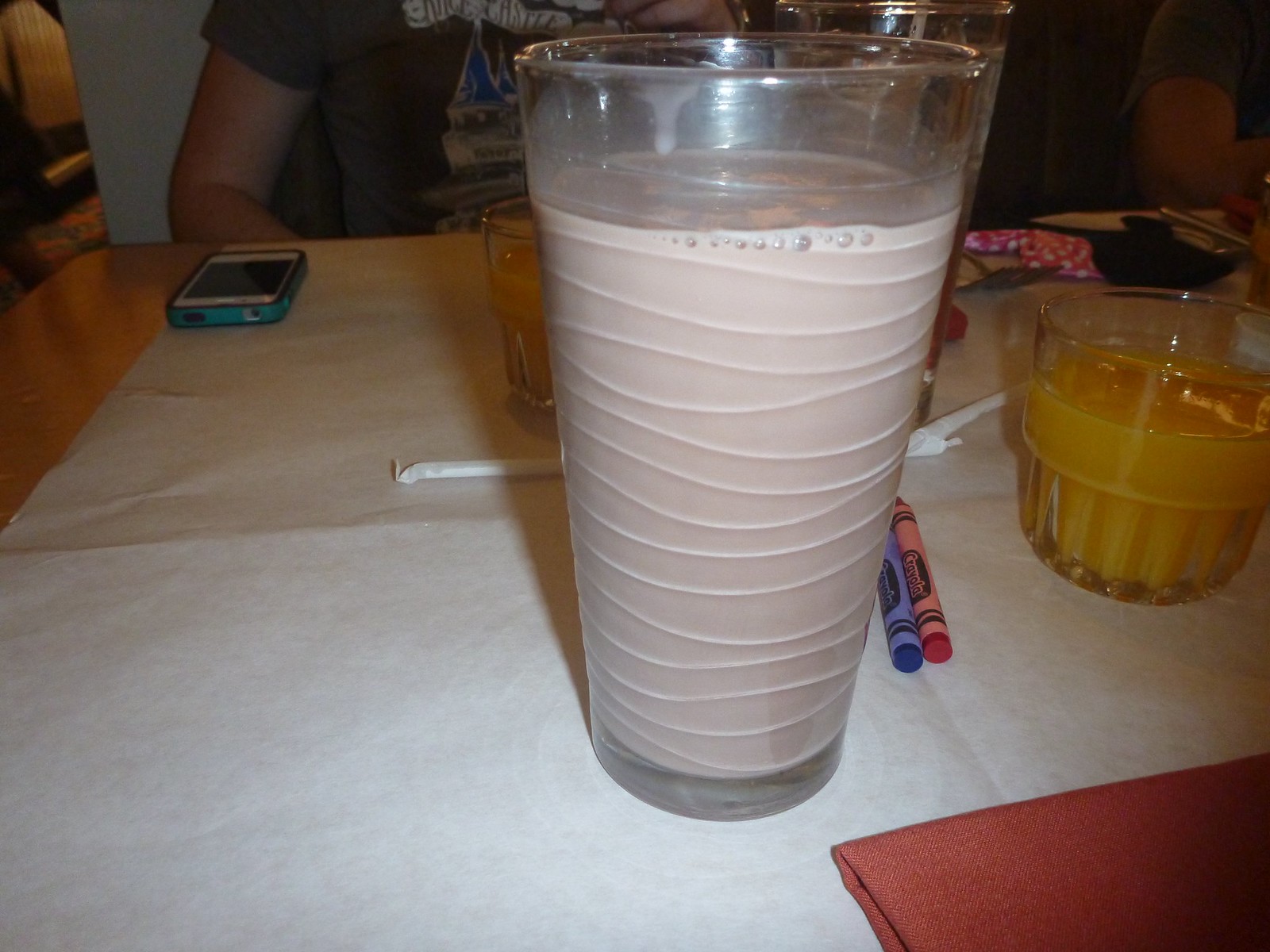The image showcases a cluttered scene on a table largely draped in white paper. Dominating the foreground is a tall clear glass filled with light brown chocolate milk, distinguished by its wavy horizontal lines. Adjacent to it on the right, sit two colorful Crayola crayons, one blue and one red. A short glass containing orange juice, identifiable by its ribbed texture, is positioned further right, alongside another similar glass behind the milk. Two straws lie horizontally behind the tall glass. In the lower right corner, a folded brown napkin is visible. Towards the rear of the table, an older model iPhone in a turquoise case rests near a bent arm clad in a black graphic t-shirt, indicating the presence of a person partially within the frame. On the far right, another individual's elbow and sleeve make an appearance.